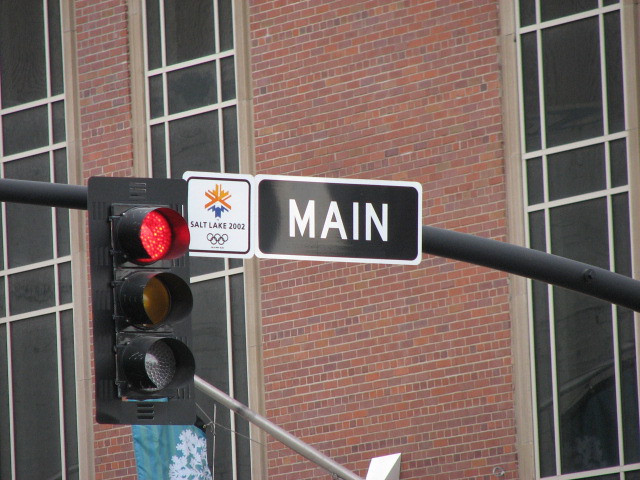This photograph, taken outside during the day, captures an urban scene with a notable focus on a traffic signal and its surrounding elements. The traffic light, mounted on a thick black steel pole curved outward, displays a lit red light at the top, with an unlit yellow light in the middle and an unlit clear light at the bottom – possibly indicating a turn signal. Adjacent to the traffic light, a sign features "Maine" in white letters on a black rectangular background with a white border. Beside it is another sign with a yellow and blue icon that reads "Salt Lake 2002" accompanied by the Olympic rings.

In the background, a distinctive building with a mixture of maroon, orange, light brown, and dark red bricks stands tall. The building's façade includes large, rectangular black-tinted windows, accentuated with white vertical and horizontal bracing. The building's windows are bordered by accent bricks in a tan color. Additionally, a silver trapezoidal structure attaches to a large silver pole that extends outward, displaying a blue flag with a white floral or snowflake pattern. This detailed and vibrant photograph appears to be set in Salt Lake City, with references to the 2002 Winter Olympics adding a historical layer to the urban backdrop.